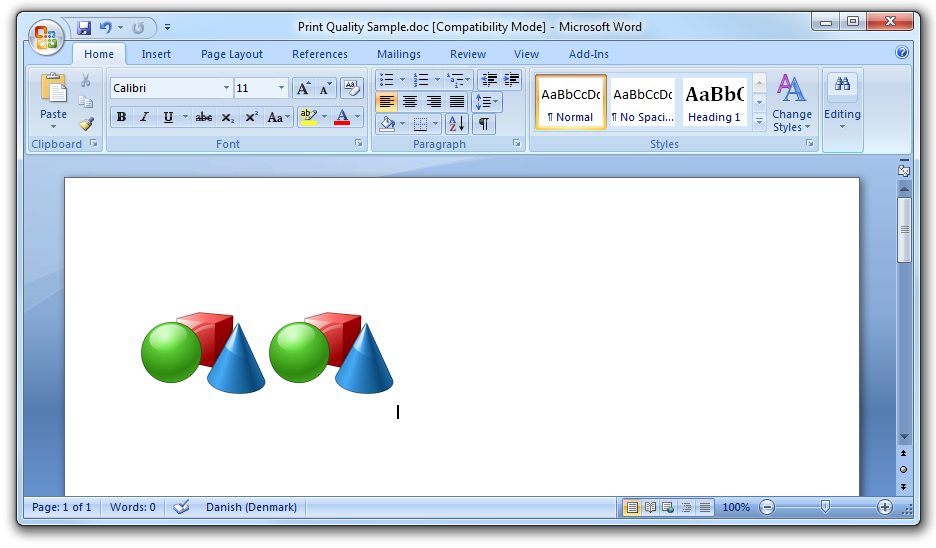This is a screenshot of a Microsoft Word document named "printqualitysample.doc" in compatibility mode. The Word window features a light bluish theme, with the Home tab active and tabs for Insert, Page Layout, References, Mailings, Review, View, and Add-ins visible. The font selected is Calibri, size 11, with typical formatting options like bold, italic, and underline. In the top left corner, the old Windows logo is visible, and a red X is present in the upper right for closing the program. The document displays no text but contains two identical images side by side on the left half of the page. Each image shows a green sphere, a red cube behind and to the right of the sphere, and a blue cone in front of and to the right of the cube.